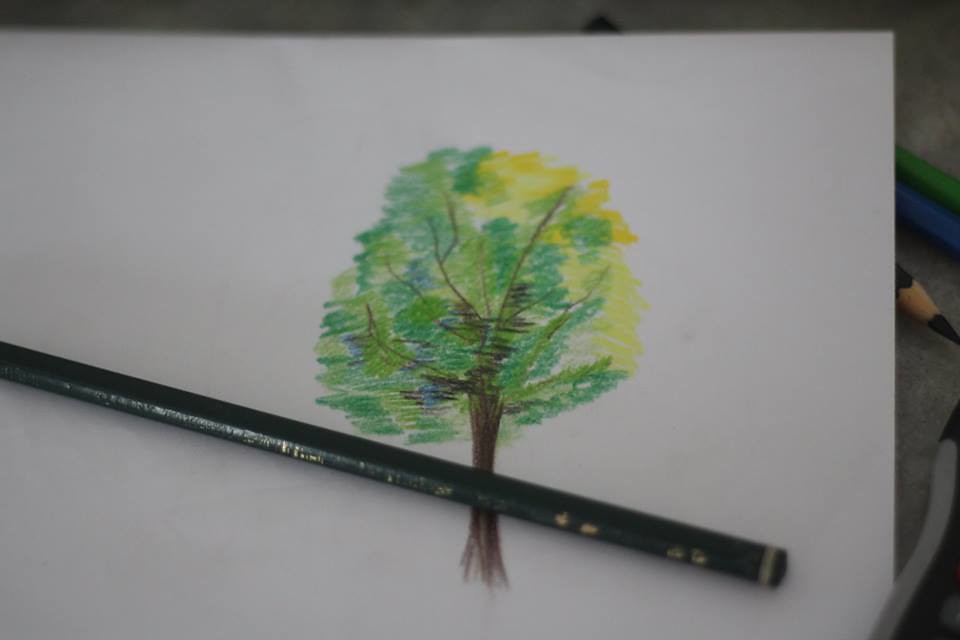This image is a landscape-oriented photograph of a colorful tree drawing on a white sheet of paper. The drawing, created with colored pencils, depicts a tree with a strong brown trunk and various shades of green and yellow in its foliage. The leaves appear to be scribbled on, using hues like hunter green, pea green, light green, and shades of yellow ranging from pale to orangish yellow. The branches, drawn in brown, contribute to the detailed shading of the tree.

Prominently, a large colored pencil, with the characteristic black exterior of the brand, lies across the drawing from the left to the bottom right corner, covering part of the tree. The background is gray, featuring three colored pencils—a green one, a blue one, and a black one—scattered around. Additionally, there is an unidentified object in the bottom right corner, possibly plastic. The overall scene showcases a vibrant yet somewhat scribbled representation of a tree in full bloom.